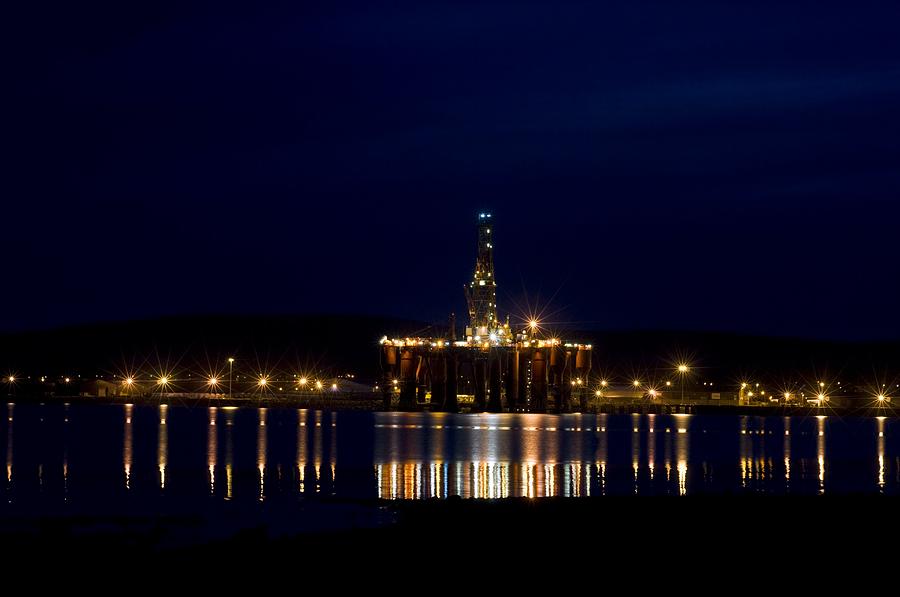The image depicts a nighttime view of a large oil rig situated along the water's edge in a bay. The photograph is rectangular, with the width being twice the height. The sky in the upper half transitions from dark blue to black and purple, indicating the capture was taken at night. The scene is visible from a shore that outlines the bottom of the photograph, giving way to a reflective, black body of water. The oil rig, the focal point of the image, is supported by multiple large orange-painted pillars and features a flat platform with a tall, single spire of metal framework extending upwards from its center. Numerous lights are scattered across the top of the rig, with additional bright yellow lights from street lamps flanking either side. The ambient lights cast shimmering reflections off the water, but no people or cars are visible in the scene.